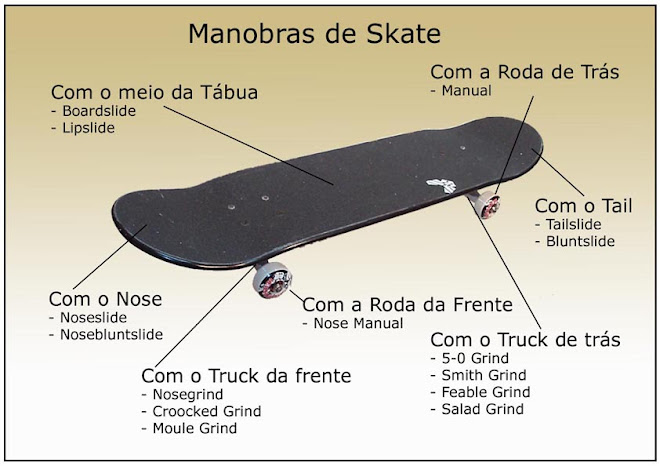The image features a detailed diagram of a skateboard set against a gradient background that transitions from tan at the top to off-white at the bottom. The skateboard, a central focal point, is black with white wheels adorned with black and red accents. The text, in Portuguese, begins at the top with the phrase "Manobras de Skate," indicating various skateboard maneuvers. Numerous arrows dissect the skateboard, identifying its components and corresponding tricks: the top deck, lip, trucks, and wheels. Specific tricks listed include nose manual, forward slide, lip slide, tail slide, blunt slide, nose slide, and five grind variations such as 5-0 grind, smith grind, and feeble grind. The diagram's instructional format, detailing both the skateboard's parts and associated tricks, suggests it might serve educational purposes, possibly sourced from a PowerPoint presentation, a book, or a sports store manual.